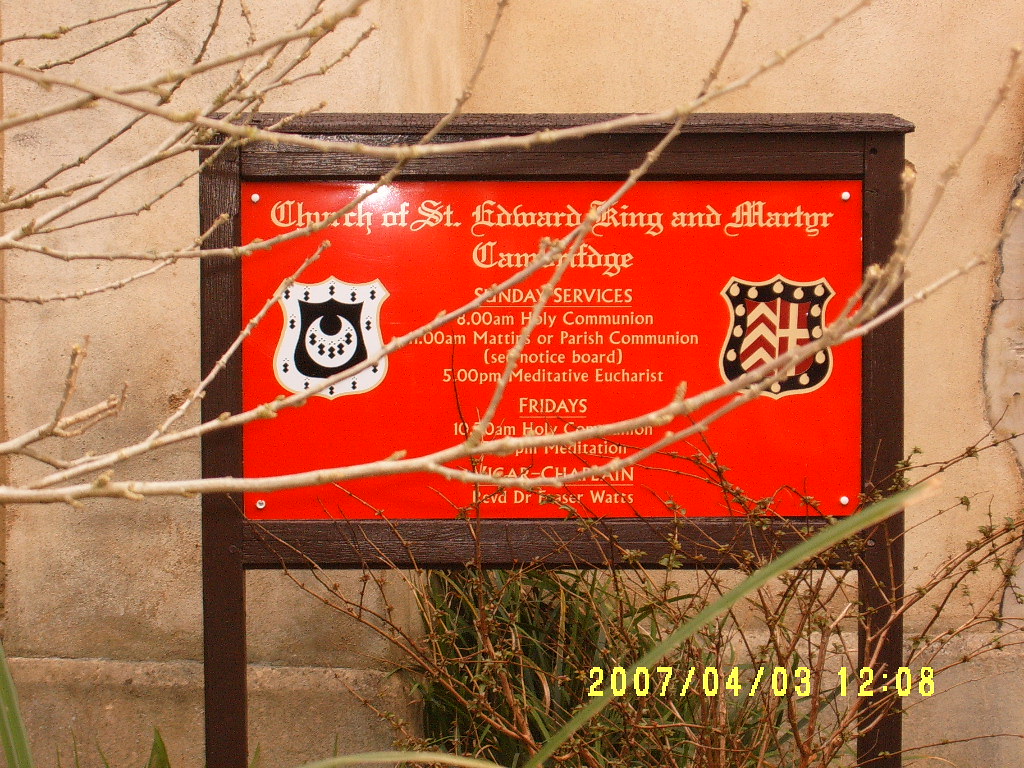In this image, a central red wooden sign stands prominently outdoors against a tan concrete wall bathed in daylight. The sign reads "Church of St. Edward, King and Martyr, Cambridge" and provides details of Sunday services: "8am, Holy Communion, 11am, Matins or Parish Communion, See Notice Board, 5pm, Meditative Eucharist." Some of the text is partially obscured by tree branches. On either side of the sign are two shields: the left one features white with black diamonds and the middle shows a black symbol resembling an upside-down moon; the right shield depicts more intricate designs in blue, off-white, and dark red. The scene is further detailed with grass and brush at the bottom, and the date "2007-04-03 12:08" is displayed in the bottom right corner of the image. This detailed capture emphasizes the historical and communal significance of the church setting.